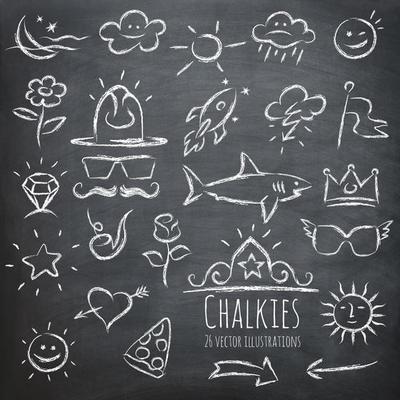The image depicts a black chalkboard with a white, chalky haze, indicative of numerous writings and erasures over time. It serves as a backdrop for 26 white chalk illustrations, titled "Chalky's 26 Vector Illustrations," as noted in the bottom right corner beneath a small drawing of a princess crown. The whimsical collection includes an array of simple yet charming drawings, such as a crescent moon accompanied by stars, a cloud with a smiley face, a basic sun with radiating lines, a rainy cloud with a sad face, a winking sun, a flower, a hat, a rocket ship, lightning, a flag, a diamond, sunglasses, a shark, a piece of pizza, a heart with an arrow, an Aztec-style sun, and more. Each illustration showcases the playful use of chalk, capturing the essence of casual yet creative doodling on a classic chalkboard backdrop.